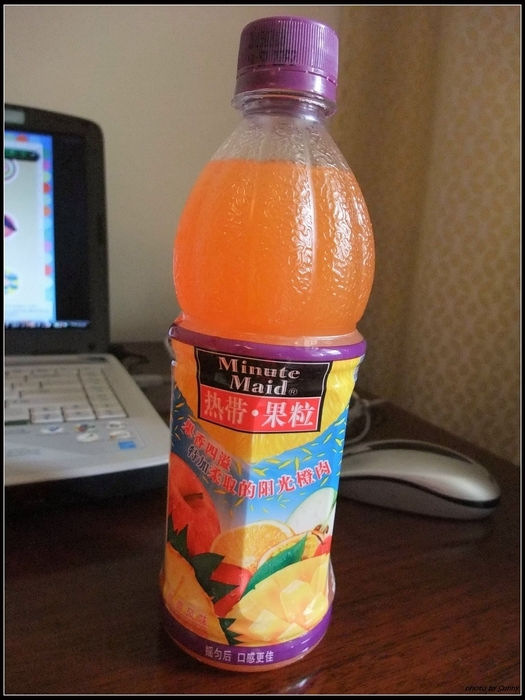This detailed image features a clear plastic bottle of Minute Maid juice with a distinct purple cap, standing upright on a dark brown table. The bottle's label prominently displays the words "Minute Maid" in white against a black background, surrounded by colorful designs. The label is accented with shades of red, orange, yellow, blue, and green, and decorated with images of various fruits such as apple, mango, pineapple, and a baby cherry at the bottom. Asian text is visible on the label beneath the "Minute Maid" branding.

The juice itself is orange in color. The surroundings include an open laptop with a gray keyboard on the left, its screen illuminated with blue hues, and a silver mouse to the right. The background of the scene is partly filled with a wall on the left side and a yellow-and-white curtain on the right. The bottle is positioned centrally, creating a focal point amidst the additional elements like the gray cord of the mouse running behind it.